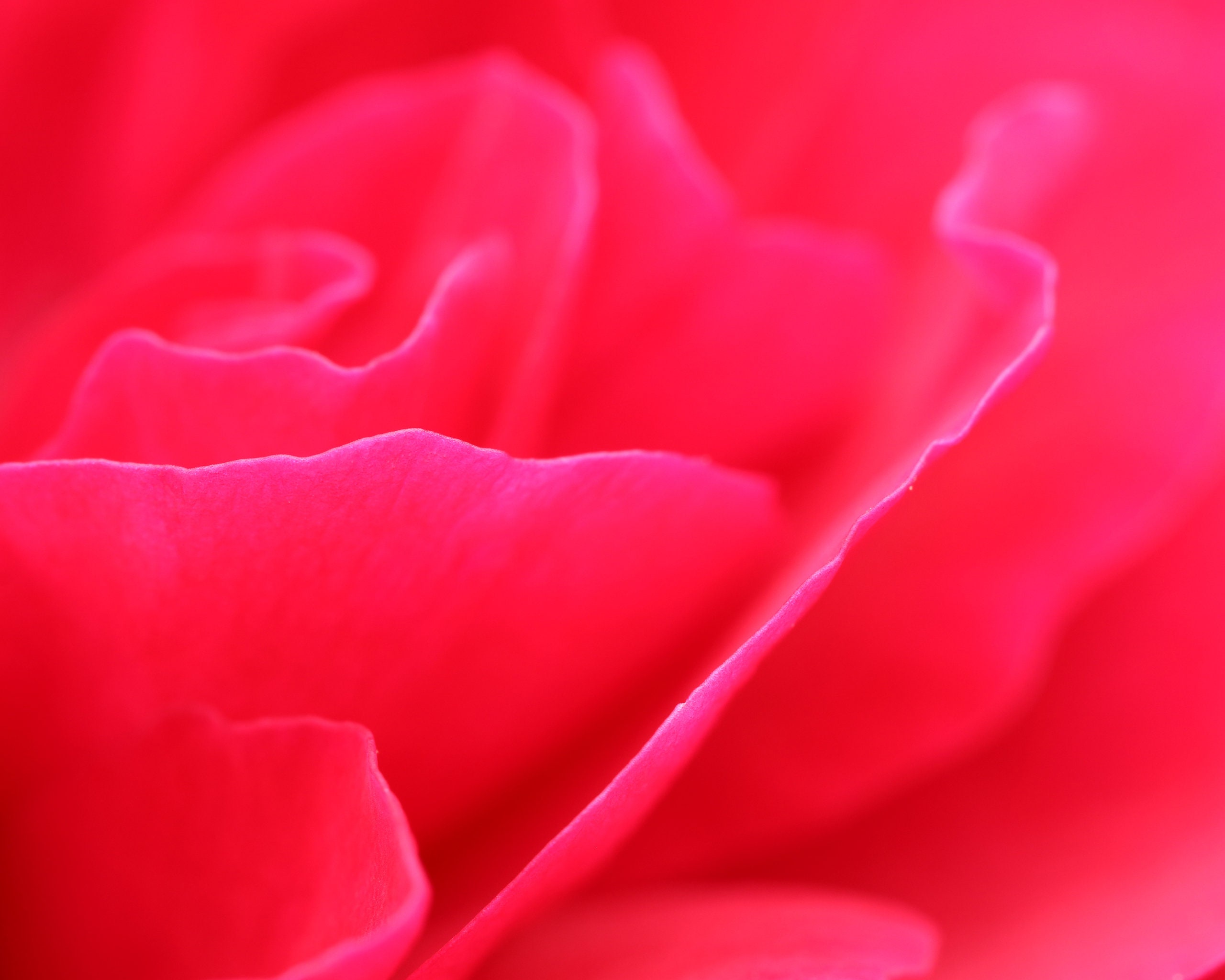This image showcases a close-up view of the intricately detailed petals of a rose. The petals display a stunning gradient of colors, ranging from vibrant red and hot pink to lighter pinks and even hints of light purple at the edges. The composition highlights the ruffled, wavy texture of the petals, which arrange themselves in a captivating, somewhat unorthodox spiral. The foreground of the image is exceptionally sharp, showing off the elegant curvature and delicate shadows of the petals, while the background gently blurs, emphasizing the depth of field. Reflections of light accentuate the petal edges, giving an almost luminescent quality to the white highlights. This detailed and vividly colored photograph artfully captures the natural beauty and complex structure of the rose.